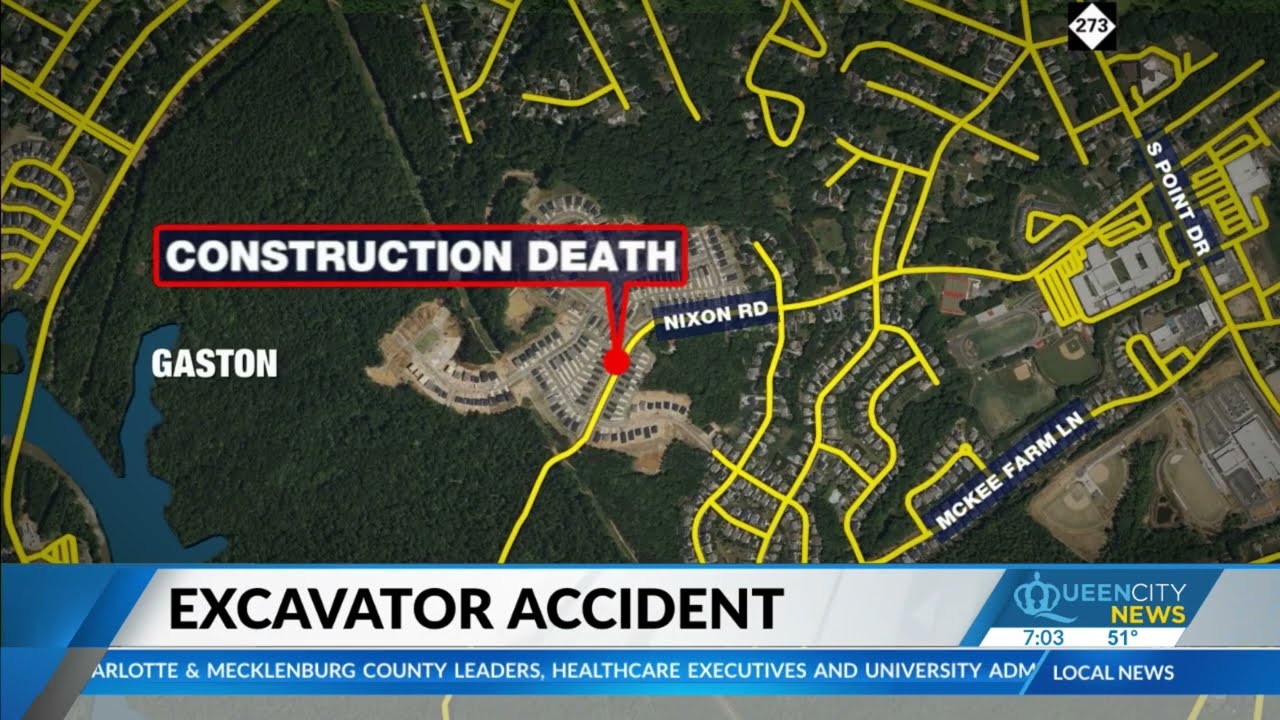The image is a video capture from a local TV newscast titled "Queen City News," showing an aerial map of a community in Charlotte, North Carolina. Text at the bottom identifies an "Excavator Accident" and features a news ticker mentioning "Charlotte and Mecklenburg County leaders, healthcare executives, and university administrators." A highlighted yellow road network prominently displays Nixon Road, where a "Construction Death" is pinpointed within an industrial complex. The map also identifies other major roads such as South Point Drive (labeled Route 273) and McKee Farm Lane leading into Three Point Drive. The area, possibly Gaston, appears on the left with suburban housing, verdant trees, and a body of water. The map and newscast overlay collectively highlight the accident location and offer detailed geographical context, further marked by a red dot and accompanying text. The time and temperature, "7:03 and 51 degrees," are also displayed.